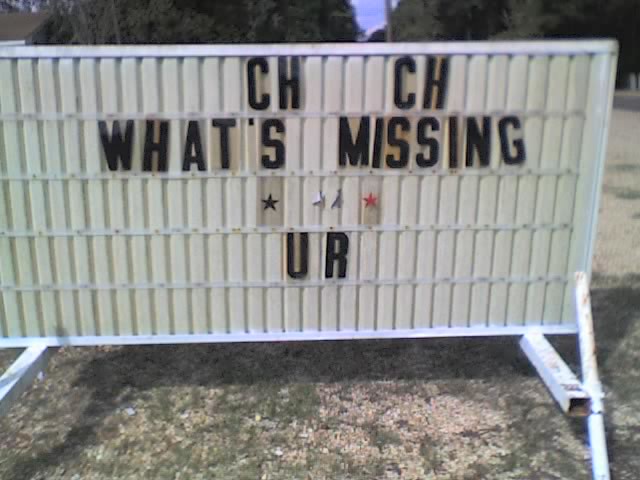A detailed, realistic photo showcases a white metal sign standing in a somewhat neglected parking lot. In the foreground, the ground beneath the sign is a mixture of gravel and overgrown grass. The parking lot, positioned behind the sign, displays visible cracks filled with tufts of grass, hinting at its disrepair. Beyond the lot, a backdrop of trees frames a small sliver of blue sky, suggesting it is daytime. Nestled among the trees is a telephone pole, and to the left, the brown roof of a house peeks through the foliage. The white metal sign features a top border and several rows designed for removable letters. The top row spells out "CHCH," followed by a second row asking "what's missing." The third row displays two stars, and the fourth row reveals the letters "U" and "R." This meticulous arrangement of letters draws the viewer's attention, prompting them to fill in the blanks and engage with the message conveyed.